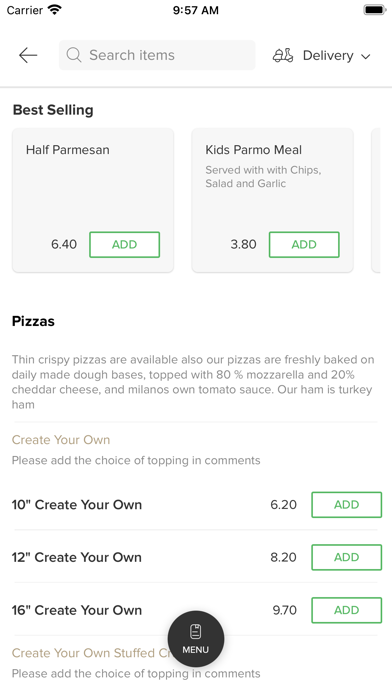A detailed screenshot from the Milano's Pizza app on a smartphone. The status bar at the top shows full Wi-Fi signal, the current time (9:57 AM), and a fully charged battery.

The app interface starts with a gray search bar reading "Search items" on the left and "Delivery" on the right. Directly below, the text highlights "Best Selling" menu items:

- **Half Parmesan** for $6.40.
- **Kids Parmo Meal** served with chips, salad, and garlic for $3.80.

Both items have small advertisement icons associated with them.

Following the best sellers section is the "Pizzas" category which emphasizes that their pizzas are made with thin, crispy bases and freshly baked daily. They use a blend of 80% mozzarella and 20% cheddar cheese, paired with Milano's signature tomato sauce. It's noted that their ham is turkey ham.

Next is the "Create Your Own" section, encouraging users to specify their topping choices in the comments:
- **10-inch Create Your Own** for $6.20,
- **12-inch Create Your Own** for $8.20,
- **16-inch Create Your Own** for $9.70.

In the middle of the screen is a round menu icon, beneath which it says "Create Your Own Stuffed Crust," again asking for topping choices to be added in comments.

The overall impression confirms this screenshot details the ordering process for Milano's Pizza via their dedicated app.